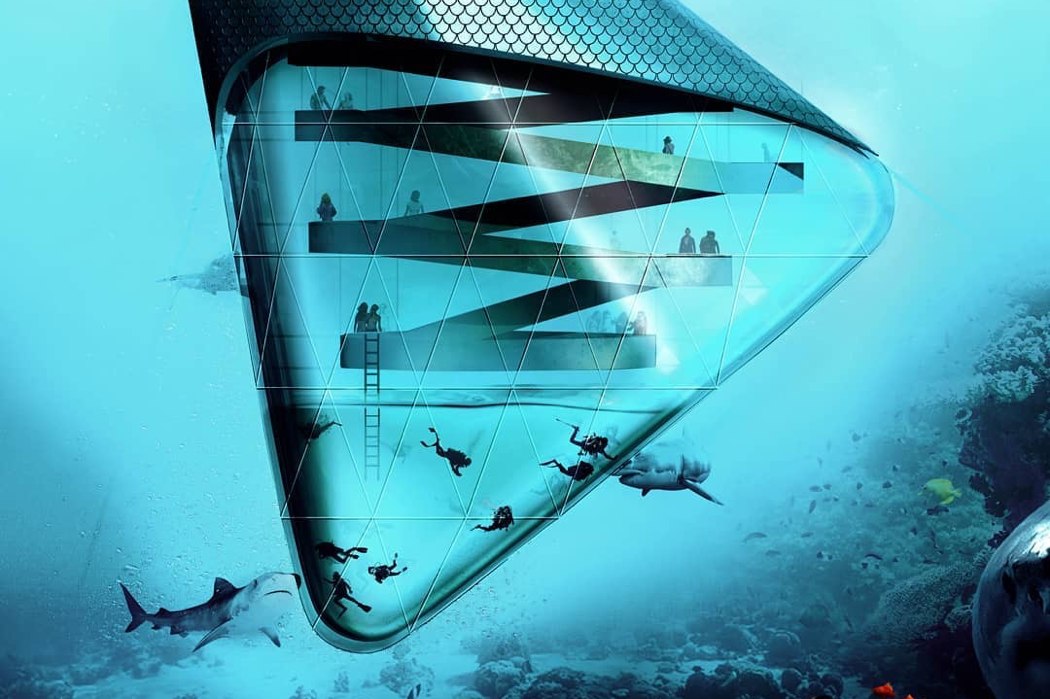This detailed digital art depicts an imaginative underwater scene featuring a futuristic glass submarine or underwater structure in the shape of a large, unconventional vessel. Positioned in the lower left of the image is one of three observable sharks, while the ocean floor beneath the scene is strewn with rocks and possibly submerged statues or large plants on the far right. In the center of the composition, a massive, intricately designed glass contraption hosts miniature figures of people, some walking along zigzagging platforms and walkways. The structure includes a ladder cascading downwards into the depths, where more individuals, donned in underwater suits with flipper feet, are seen exploring and taking photos. Shafts of light penetrate the ocean, illuminating the area and highlighting a yellow fish situated in the middle right. The overall atmosphere suggests a conceptual and futuristic underwater exploration or observation habitat, with features that appear both surreal and technologically advanced.